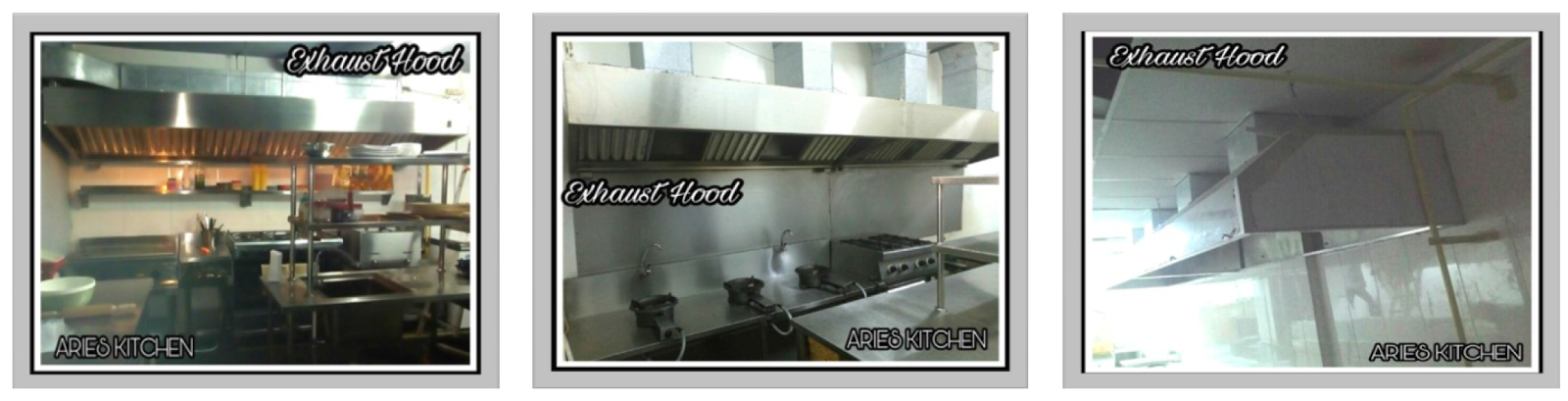In a composite image featuring three adjacent photographs of commercial kitchens, each framed by a thick gray border, the primary focus is on the sleek, metallic exhaust hoods. The leftmost image showcases a commercial kitchen with ambient orange lighting beneath the exhaust hood, emphasizing the functional workspace which includes a service cart and countertops. The text "Exhaust Hood" in small cursive is situated at the top right, while "Aries Kitchen" is inscribed in the bottom left corner.

The central photograph also features a commercial kitchen, highlighting a long exhaust hood with four large vents extending to the ceiling. Below the hood, there are deep fryers and a stovetop, and part of a service table is visible in the foreground. Similar to the first image, it includes the cursive "Exhaust Hood" on the middle left and "Aries Kitchen" in white text at the bottom right.

The third image offers a closer look, focusing on the exhaust hood with three distinct vents trailing up to the ceiling. A bright background reveals reflections from a nearby window, adding a touch of contrast. Consistent with the previous images, it features the cursive "Exhaust Hood" in the top left and "Aries Kitchen" in white text at the bottom right.

Together, these images provide a detailed and consistent visual representation of exhaust hoods in commercial kitchen settings, accentuated by the recurring brand identity of "Aries Kitchen."